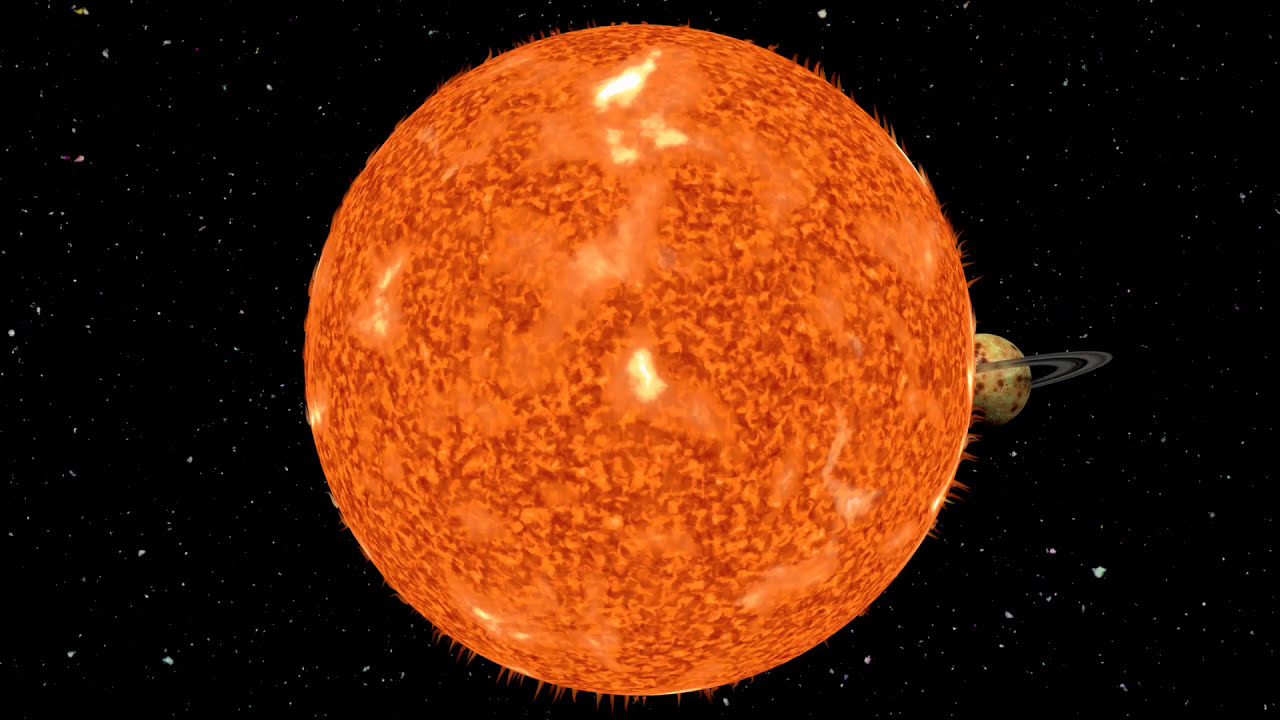This computer-generated image, seemingly produced through CGI and possibly viewed through an infrared telescope, features a prominent depiction of the Sun amidst a black backdrop dotted with stars. The Sun takes center stage as a large, medium-orange sphere with darker orange splotches and white-orange clouds scattered across its surface. It's encircled by numerous tiny solar flares or gas spikes radiating outward from its edges. To the right of the Sun, there's a Saturn-like planet, distinguishable by its brownish-yellow hue and ring system, though its color and characteristics differ slightly from the actual Saturn. This planet appears unusually close to the Sun in the image, suggesting an artistic reinterpretation rather than a factual celestial arrangement. The intricate details of the Sun's surface and the surrounding stars add a layer of realism, though the scene as a whole remains a beautifully constructed piece of digital artistry.